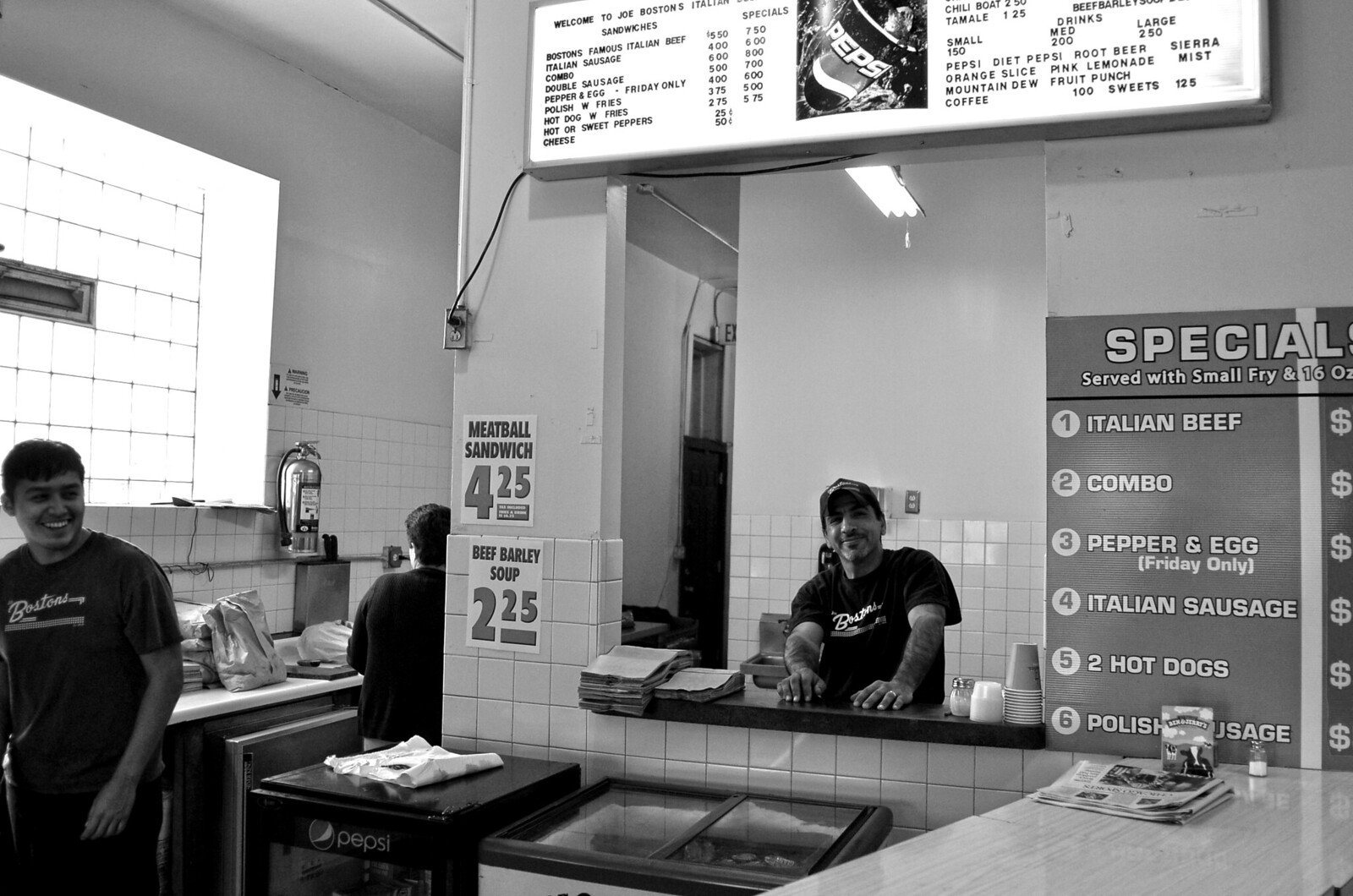This black-and-white photo captures the bustling interior of "Joe Boston's Italian Sandwiches," a fast food restaurant specializing in Italian fare. Front and center is a cheerful man behind the counter, sporting a t-shirt and a baseball cap emblazoned with the company's logo. To the left, another man, also in a company t-shirt, stands smiling. Behind him, a woman faces away from the camera, adding to the lively atmosphere.

The left side of the image is bathed in natural light from a window, illuminating the scene. Above the main counter hangs a large, backlit menu sign displaying a variety of offerings and prices. Items featured include "Boston's Famous Italian Beef" for $5.50 and $7.50, Italian sausage for $4.00 and $5.00, and specials like the Polish sausage combo for $4.00 and $8.00, along with Friday-only pepper and egg sandwiches. Additional items listed are meatball sandwiches for $4.25, beef and barley soup for $2.25, and a range of drinks, including Pepsi products.

To the left of the man at the counter is a smaller sign highlighting a meatball sandwich and beef and barley soup, with a fluorescent light overhead casting a bright ambiance. Below the counter, an iced soda cart holds various beverages, adding a touch of practicality to the setup. The detailed layout and smiling staff invite patrons into this classic eatery known for its hearty Italian-American dishes.